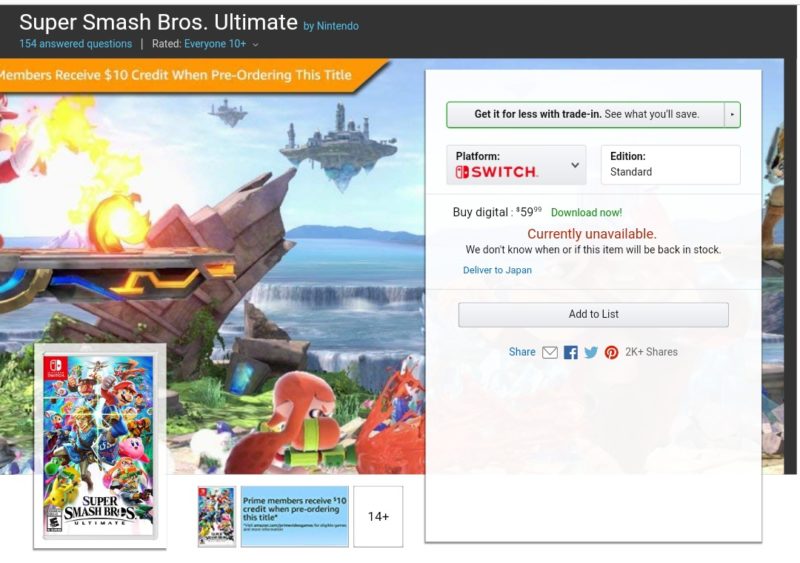Screenshot from the video game "Super Smash Bros. Ultimate," displayed on a website. The top section features a black horizontal rectangle with the game's title, "Super Smash Bros. Ultimate," in white text. The words "By Nintendo" appear next to it in blue print. Beneath the black bar is an orange rectangle that spans the width of the screen, bearing the message: "Members receive $10 credit when pre-ordering this title" in bold text.

Descending down the page, the image transitions into a vibrant depiction of the Super Smash Bros. world. The background is an intricate blend of floating islands with airships scattered throughout the sky. A majestic waterfall cascades from a distant peak, while fiery projectiles rain down from the upper left corner, striking a curving rock formation. Prominently displayed in the scene is a character resembling a monkey with distinct green stripes on its face.

In the lower part of the image, a box art of the Super Smash Bros. Ultimate game for the Nintendo Switch is shown. The box indicates that the game is currently unavailable, highlighted in red text.